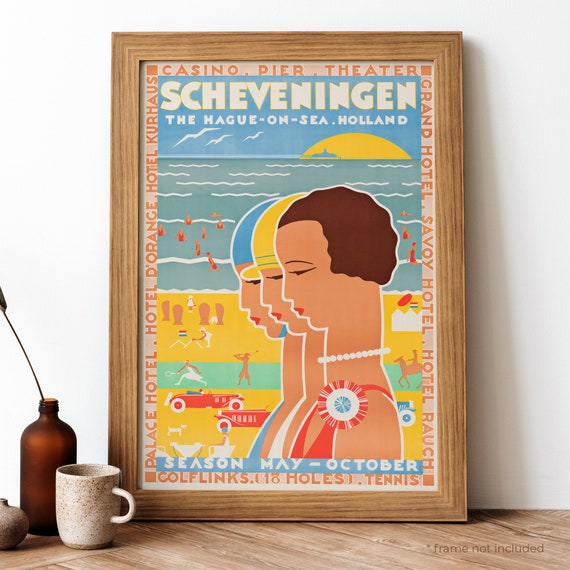The photograph depicts a vintage-looking, art deco poster encased in a light wooden frame, leaning against a stark white wall and positioned on a diagonally planked wooden table. The poster, titled "Scheveningen, The Hag on Sea, Holland," measures approximately 2.5 feet tall by 2 feet wide. It advertises a range of attractions for the season running from May to October, including the Casino Pier Theater, Grand Hotel, Savoy Hotel, Golf Links (with 18 holes), Tennis, Palace Hotel, Hotel de Oranje, and Hotel Kurhaus, all listed in red and white text around the border. 

The central illustration features a beach scene at sunset with a blue sky adorned with white birds and ocean waves lapping at the shore. People are depicted enjoying various beach activities, and several vintage cars, evocative of the 1920s, line the background. Three women, their faces in profile, dominate the foreground. The foremost woman has short brown hair, wears a pearl necklace, a red sleeveless vest, and what appears to be a badge on her shoulder. The other two women, positioned in depth, don white and blue outfits with corresponding headgears.

To the left of the poster, on the table, sit a white coffee cup, a brown glass jar containing a leafy stem, and a small decorative item. The entire scene captures a blend of simple, elegant nostalgia and creative graphical design.